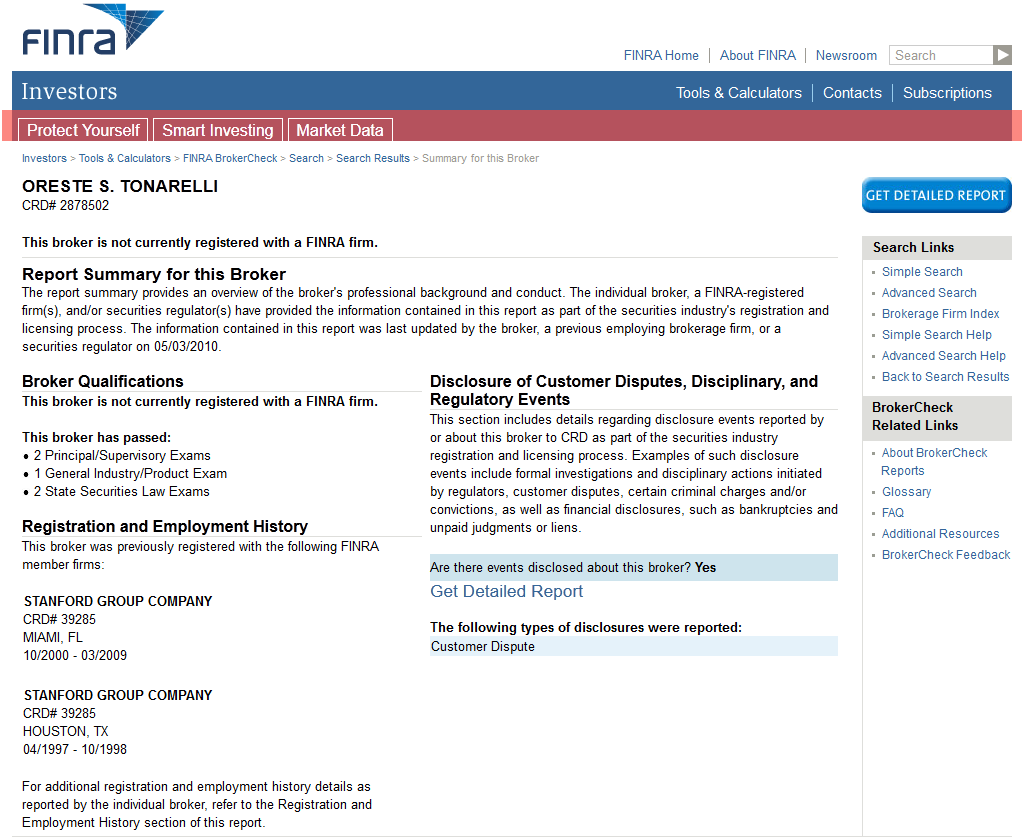The image displays a webpage from Fenra, a financial regulatory authority. In the upper right-hand corner is the Fenra logo accompanied by the text "Fenra" and an emblem that resembles two geographic graphs. The website is primarily text-based, without images. The top navigation bar includes links labeled "Fenra Home," "About Fenra," "Newsroom," and a search box.

A secondary navigation bar is present; on the far left, it lists "Investors," and on the far right, "Tools and Calculators," "Contacts," and "Subscriptions." Below this navigation bar is a red strap that houses stylized tabs labeled "Protect Yourself," "Smart Investing," and "Market Data."

The main content of the webpage provides detailed information about a specific broker. Breadcrumbs at the top of this section indicate the user is in the "Investors > Tools and Calculators > Fenra Broker Check > Search > Search Results > Summary" pathway. The broker in question is Oresti S. Tonarelli, with a corresponding CRD number indicating he is not currently registered with a Fenra firm. The report summary includes sections on qualifications, disclosure information, registration, and employment history. It notes that Oresti S. Tonarelli was employed by the Stanford Group Company from 1997 to 1998 and from 2000 to 2009.